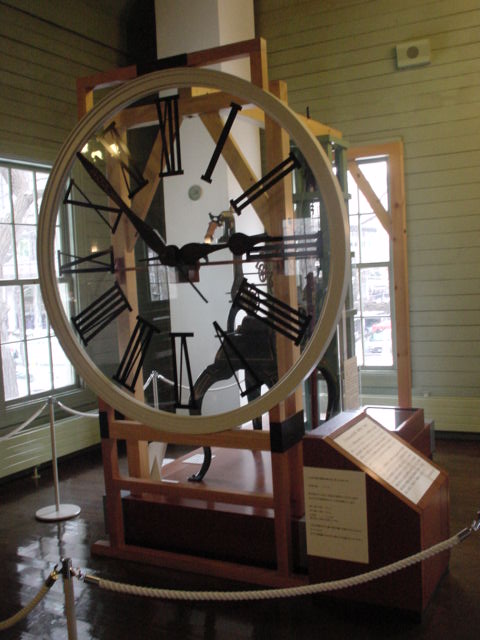In a well-lit room adorned with light green shiplap walls, a colossal wooden stylized clock face commands attention. The room is brightened by large white windows, each comprising twelve glass panes that allow natural light to pour in. Positioned prominently in the room, the clock is encircled by a museum rope barrier, supported by white stanchions, that demarcates its space.

The clock itself features an elegant, light-colored wooden frame, hosting bold black Roman numerals that appear to float against the backdrop from 1 to 12. Striking black wrought iron hands add to the clock's grandeur, poised to mark time. Behind the clock, a wooden framework supports a sophisticated mechanism, crafted from wrought iron and metal, designed to operate the clock hands.

Anchoring the display, the clock and its mechanical components rest on a darker, reddish medium wood base, lending contrast and gravitas to the exhibit. Nearby, an informational stand provides contextual details about the clock, highlighted by a white sign with black text and an additional piece of paper featuring more information. To the upper right of the installation, an intercom blends into the green wall, adding a subtle touch of modernity to the otherwise historical setting.